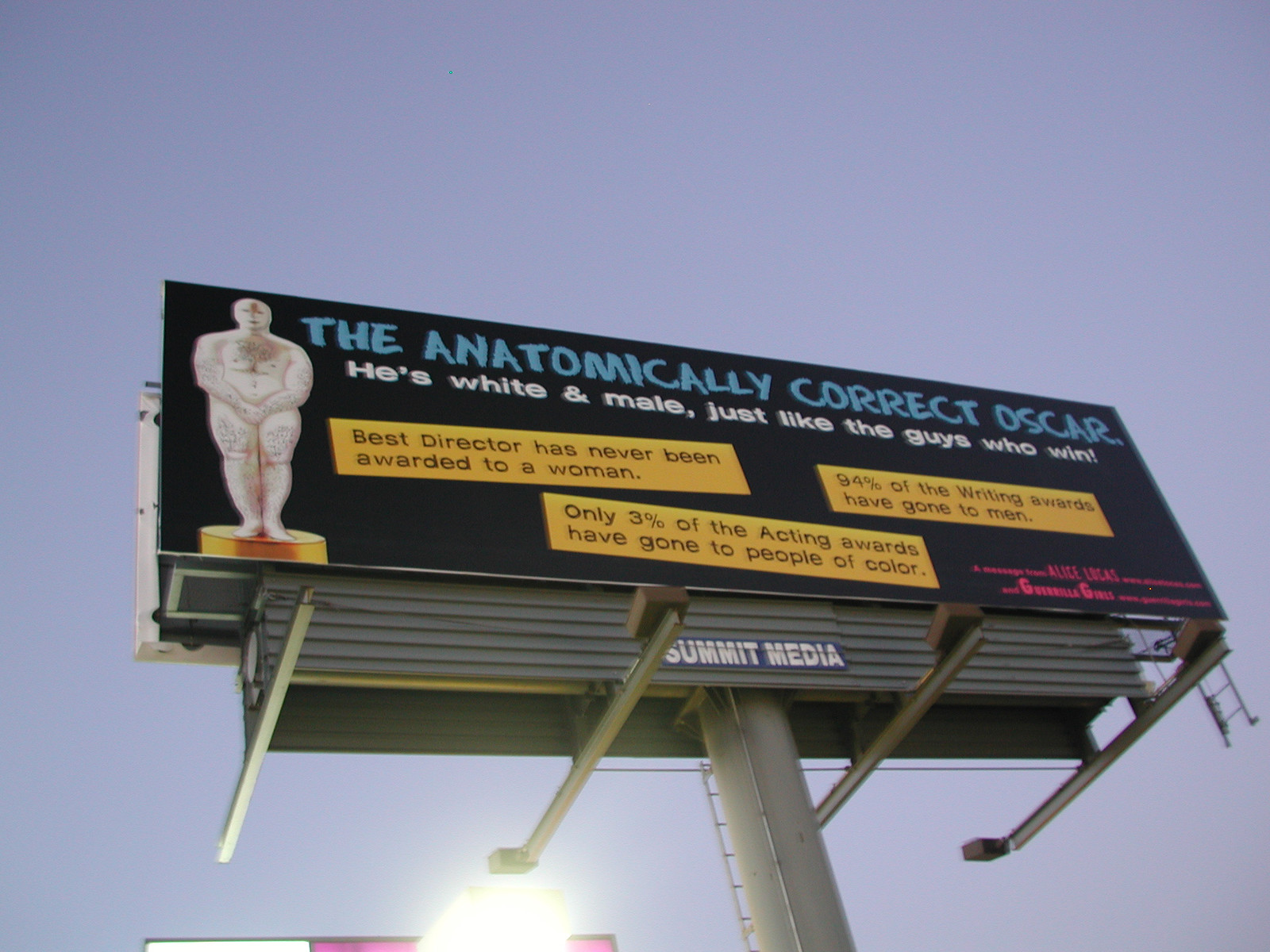The photograph captures a billboard, taken from an upward angle at ground level, emphasizing the towering presence of the sign. The billboard is predominantly black with blue text at the top, which reads, "The Anatomically Correct Oscar." Below this, white text states, "He's a white male just like the guys who win." Further down, the billboard is divided into three yellow blocks, each containing a sobering statistic: "Best Director has never been awarded to a woman", "Ninety-four percent of the writing awards have gone to men", and "Only three percent of the acting awards have gone to people of color." On the left side of the billboard, there is an image of a statue positioned on a gold pedestal. The statue, which is white and devoid of any hair, is notably portly with its private parts obscured. The messaging is clearly a critique of the lack of diversity in the Oscar awards.